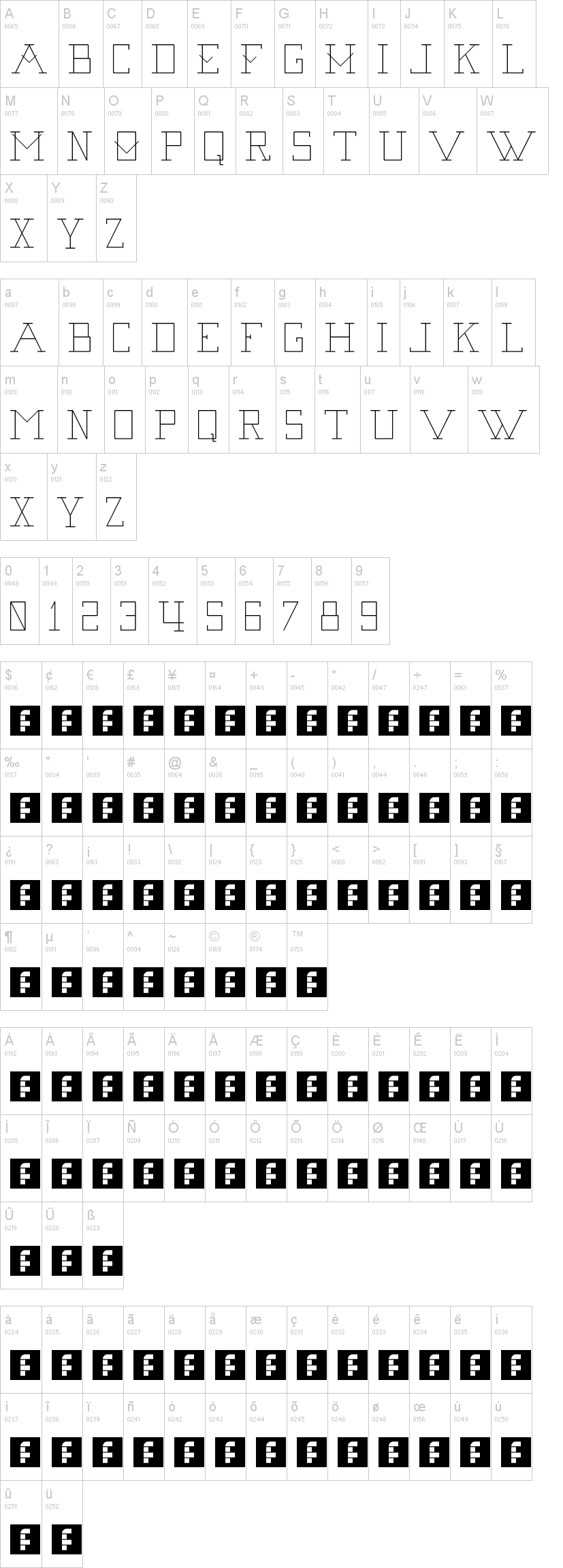The image displays a comprehensive chart of alphanumeric characters and symbols, organized into several distinct sections for clarity and reference.

**Top Section: Uppercase Letters**
1. **First Group**: A sequence of capital letters from A to L.
   - Capitals: A, B, C, D, E, F, G, H, I, J, K, L
2. **Second Group**: A continuation of capital letters from M to W.
   - Capitals: M, N, O, P, Q, R, S, T, U, V, W
3. **Third Group**: The concluding set of capital letters from X to Z.
   - Capitals: X, Y, Z

**Middle Section: Mixed Case Letters**
- This section pairs lowercase and uppercase letters within each space, with lowercase letters positioned in the top left and uppercase letters in the main area.
    - Example: (small 'a', capital 'A'), (grayed-out small 'b', capital 'B'), (small 'c', capital 'C', etc.).

**Bottom Section: Numbers and Symbols**
1. **Numbers**: Each number is shown in two styles: grayed-out and bold.
   - Sequence: 0, 1, 2, 3, 4, 5, 6, 7, 8, 9
2. **Symbols**: A variety of common and currency symbols, followed by mathematical operators.
   - Symbols: Dollar sign ($), cent (¢), euro (€), British pound (£), Japanese yen (¥), a small square (dot), plus (+), minus (-), asterisk (*), forward slash (/), division (÷), equal (=), percentage (%)
3. **Special Note**: Below each symbol, there is a unique character—a small letter 'f' accompanied by a black square.

This detailed structure ensures each set is easily distinguishable and provides a clear reference for various characters, making it useful for educational or design purposes.